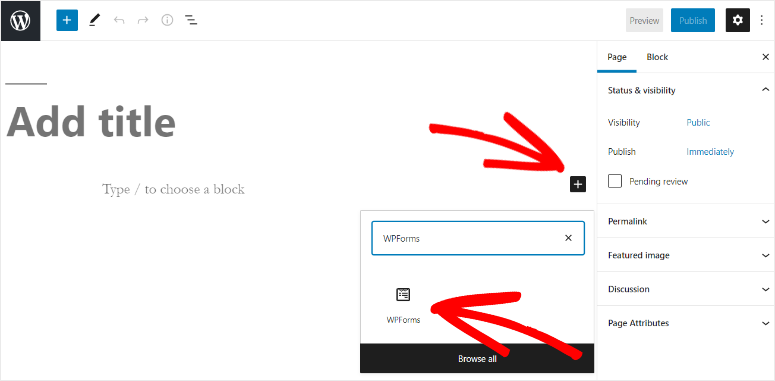The image showcases the interface of a web page, detailing the elements present in the toolbar and the sidebar. At the top-left corner, there is a black square with a white "W" inside a circle. Next to it, there is a blue square with a plus sign, followed by a pencil icon. Further to the right, there are left and right arrows, a circle with a lowercase "i" inside it, and three horizontal lines stacked diagonally. 

To the right of these icons, there is a light gray box labeled "Preview," a dark blue box labeled "Publish," and a black box with a settings gear icon. Below these elements, the interface shows the word "Page" with a dark blue underline. To the right, it says "Block" with an "X" next to it.

In the sidebar section titled "Status and Visibility," there are subsections elaborating on various attributes of the page. Under the "Visibility" subsection, a blue hyperlink labeled "Public" appears to the right. Below, the "Publish" subsection includes a blue hyperlink labeled "Immediately" to the right. There is also an unchecked checkbox with the label "Pending Review." 

A light gray horizontal line divides this section from the next, which is labeled "Permalink" and includes a drop-down menu.